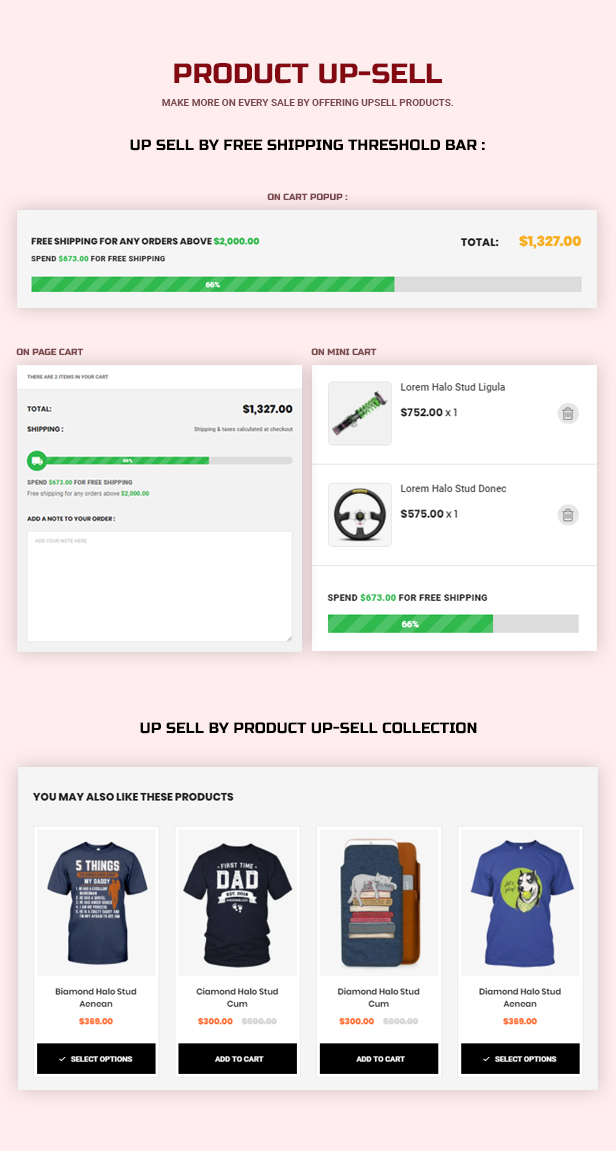A detailed screenshot of a mobile e-commerce platform showcasing a product upsell feature designed to increase sales. The site encourages merchants to boost their revenue by offering upsell products. A notable element is a "Free Shipping Threshold Bar," indicating that customers receive free shipping on orders exceeding $2,000. The current order value stands at $1,300, visually represented by a progress bar.

The interface also displays a section labeled "On Mini Cart" featuring products like the "Lorem Halo Stud." Another image depicts what appears to be an attachable driving wheel, possibly for a car or a video game setup. 

At the bottom of the screenshot, there are displayed items including t-shirts and a phone case. The overall design of the site uses a light pink background, creating a soft and inviting aesthetic. Despite the variety of elements, the layout seems somewhat complex and might require further clarity for better user understanding.